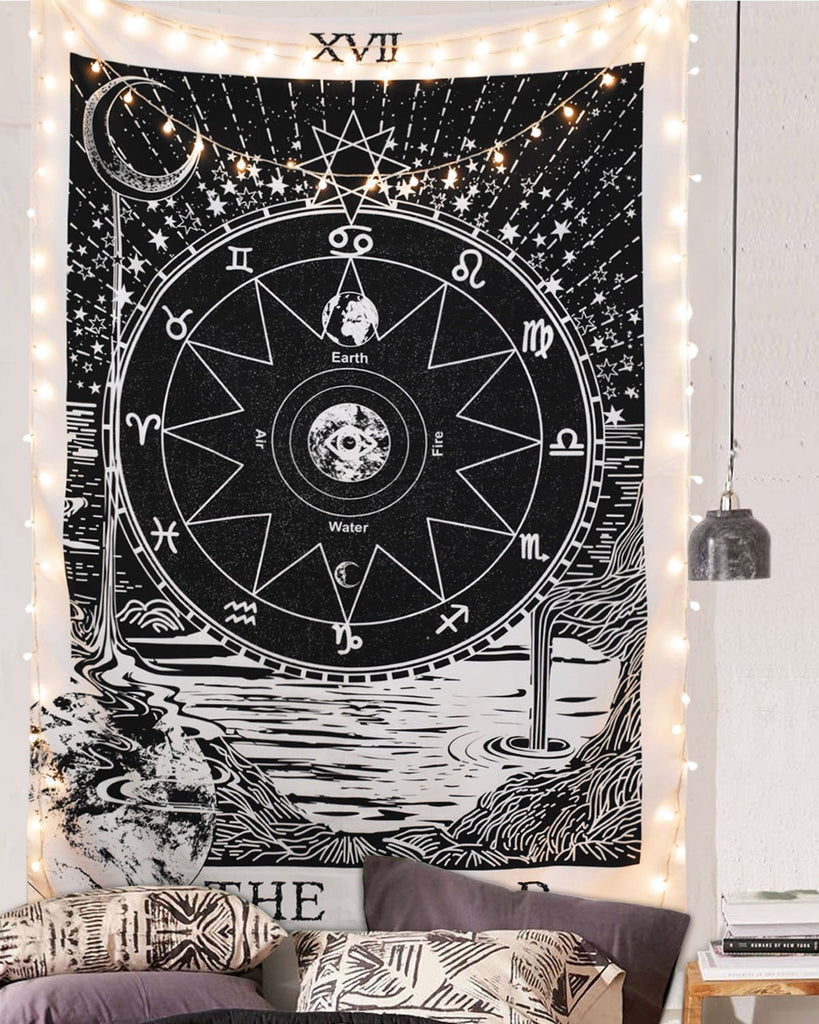This image captures a cozy and thoughtfully decorated room, details of which include a prominent black and white zodiac-themed fabric wall hanging. This tapestry showcases a large, circular design featuring various zodiac symbols positioned around the points, labeled "earth" at the top, followed by "fire," "water," and "air." Surrounding this central circle are intricate drawings including stars, landscapes with a body of water, and a moon in the upper left. Small, warm-colored string lights frame the tapestry, adding a gentle glow to the setting.

Beneath the tapestry sits a couch adorned with four decorative pillows. Two pillows showcase a beige base with black line designs, while the other two display a purple cover with additional dark gray and white patterns. To the right of the tapestry hangs a long pendant light with a gray metal shade, suspended by a wire. Adjacent to the couch, a robust wooden table holds several stacked books, enhancing the room's welcoming atmosphere. The walls of the room are a light gray, providing a subtle backdrop that highlights the intricate decor elements.